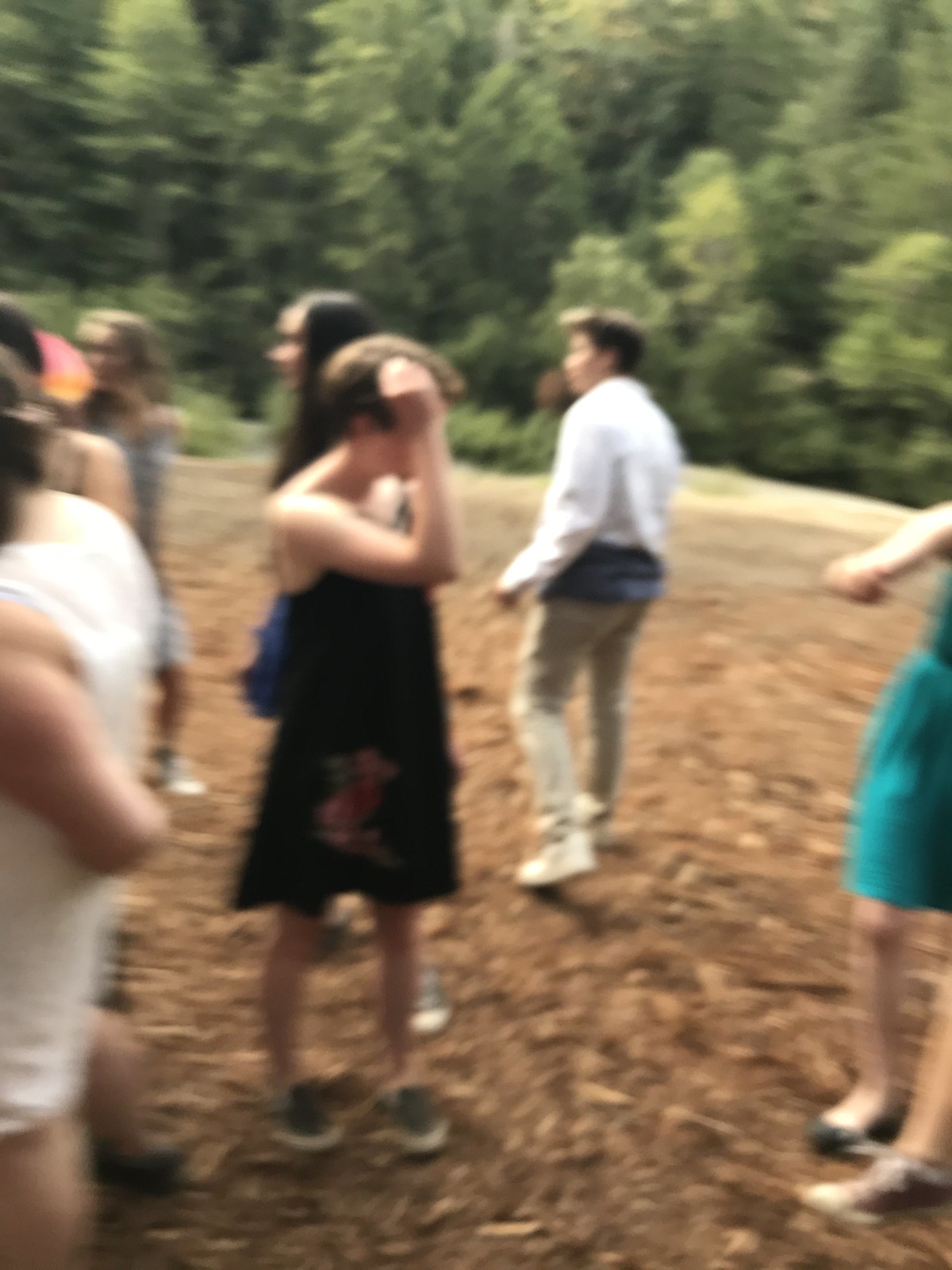In this vertically oriented, blurry color photograph, we observe a group of middle to high school-aged kids standing together on a reddish-brown dirt or mulch surface, set in an outdoor environment that appears to be a park or forest. The background is dominated by lush, tall evergreen trees that span the upper half of the image. Among the group, most individuals seem to be women dressed in various outfits, including skirts, dresses, and bare arms, indicating warm weather. Notably, there is one person in a black blouse and blue sneakers looking towards the right while the majority, including a boy in a white denim jacket, grayish khaki pants, and white sneakers, are gazing towards the left. The photograph's blurriness and wavy lines suggest it was taken while the camera was in motion, giving it a somewhat dizzying effect and making the individuals out of focus and indistinct.